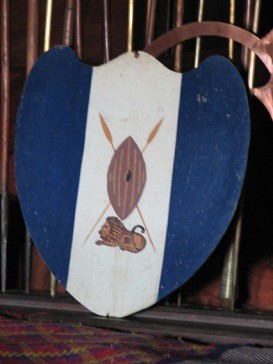The image depicts a uniquely shaped shield made of wood, resting against a dark brown wooden wall with spaces between the planks, allowing shafts of yellow light, likely from the sun, to filter through. The shield exhibits a modified heart shape; instead of the typical two curves at the top, it features a central third bump, creating a wave-like pattern. The shield is painted in a striking combination of navy blue and white, divided into three sections. The left and right sections are solid navy blue, while the middle section is white. Centered on the white section is a detailed depiction of a lion sitting on all fours with its tail raised. Above the lion, two spears crisscross, and an oval-shaped emblem is positioned at the intersection of the spears. The shield rests against a rug, contributing to the overall aesthetic of the scene.